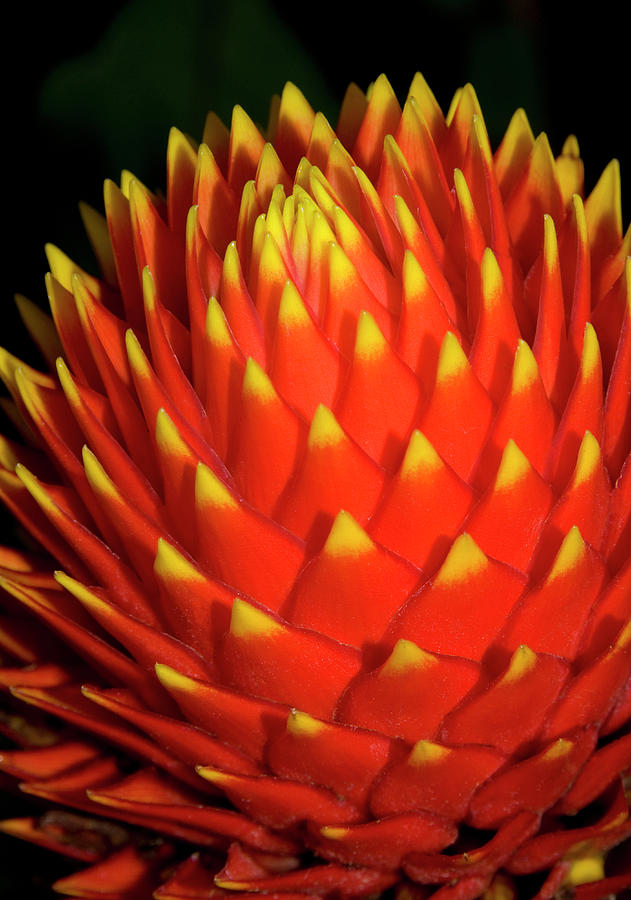The image showcases a striking and exotic bulb-like structure, possibly a fruit or tropical flower, set against a nearly black background. The object is round and densely packed with numerous triangular petals, reminiscent of a tightly compressed pine cone or a flower bud about to bloom. The petals are primarily a vibrant red-orange hue, with some petals leaning more towards red or orange shades. Each petal culminates in a sharp point, transitioning to a sunflower yellow at the tip, and slightly green at the very topmost tip. The petals are tightly clustered at the center and sparser towards the edges, where they also appear more outwardly extended and some slightly curved inward. The detailed coloration and the structural arrangement give the object an intricate, almost scale-like appearance.